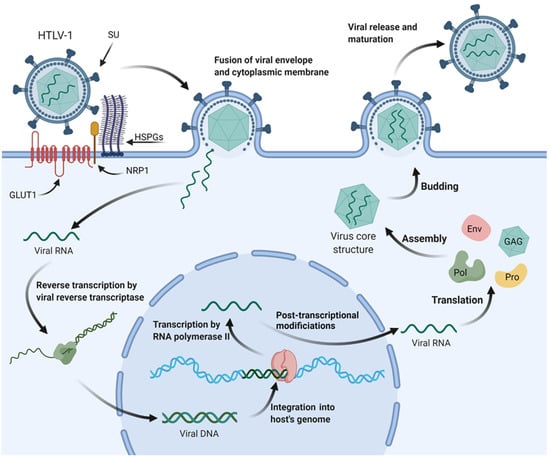This detailed diagram represents the lifecycle of the HTLV-1 virus. The image predominantly uses shades of blue with accents of pink, green, and yellow to highlight specific elements. At the top, "HTLV-1" is labeled above a depiction of the virus. The diagram illustrates several stages of the viral process:

1. **Virus Entry**: A visual representation shows the virus entering through the skin, marked by the caption "fusion of viral envelope and cytoplasmic membrane."
2. **Viral Maturation**: Adjacent illustrations depict "viral release and maturation" where the virus undergoes further development.
3. **Molecular Details**: Inside the skin depicted further are sketches of various molecules crucial for the viral lifecycle. This includes stages such as "reverse transcription by viral reverse transcriptase" where viral RNA is transcribed into DNA.
4. **Integration and Transcription**: The central part of the diagram, encircled by blue dashes, highlights "transcription by RNA polymerase" and "post-transcriptional modifications," showing how the viral DNA integrates into the host genome and begins the process of transcription to produce viral RNA.
5. **Viral Assembly**: Further stages showcase the virus core structure and the processes of "translation, assembly, and budding," representing the final steps of viral replication.

The detailed infogram not only visualizes the virus's lifecycle but also annotates various critical biochemical processes, making it highly descriptive and informative.